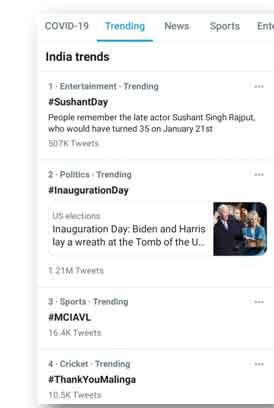**Detailed Caption:**

This image showcases a trending news dashboard from India Trends, prominently featuring various headlines and topics. At the top, the major heading is "COVID-19," indicating ongoing updates related to the pandemic. Adjacent to this is the word "TRENDING," highlighted in a vibrant blue color, emphasizing the current popular discussions. The navigation bar includes other categories like "NEWS," "SPORTS," and a truncated "ENT," likely representing "ENTERTAINMENT."

1. **Entertainment Trending:**
   - **#1**: The top entertainment trend is "Shashank Day," which is distinguished in bold black letters. This refers to a tribute to the late actor Shashank Singh Rautbud, who would have celebrated his 35th birthday on January 21st. The trend has amassed an impressive 507,000 tweets.

2. **Politics Trending:**
   - **#2**: The second trending topic in politics is "Inauguration Day," which is marked with a number sign and highlighted in black. This includes keywords related to the U.S. elections, "Inauguration Day," "Biden and Harris," and a note about a wreath-laying ceremony at the Tomb of the Unknown Soldier. An accompanying image shows President Biden with his hand raised, surrounded by others in attendance, reinforcing the significance of the event. This topic garnered 1.21 million tweets.

3. **Sports Trending:**
   - **#3**: In sports, the trend "#MCIAVL" (indicating a match between Manchester City and Aston Villa) is gaining traction with 16,400 tweets.
   - **#4**: Another sports trend is "#ThankYouMalinga," a tribute to the cricketer Lasith Malinga, highlighted in black and generating 10,500 tweets.

The overall layout features a clean, white background with mostly black text, ensuring clarity and readability. The sole image of President Biden during his inauguration adds a visual anchor to this informative snapshot of trending topics.